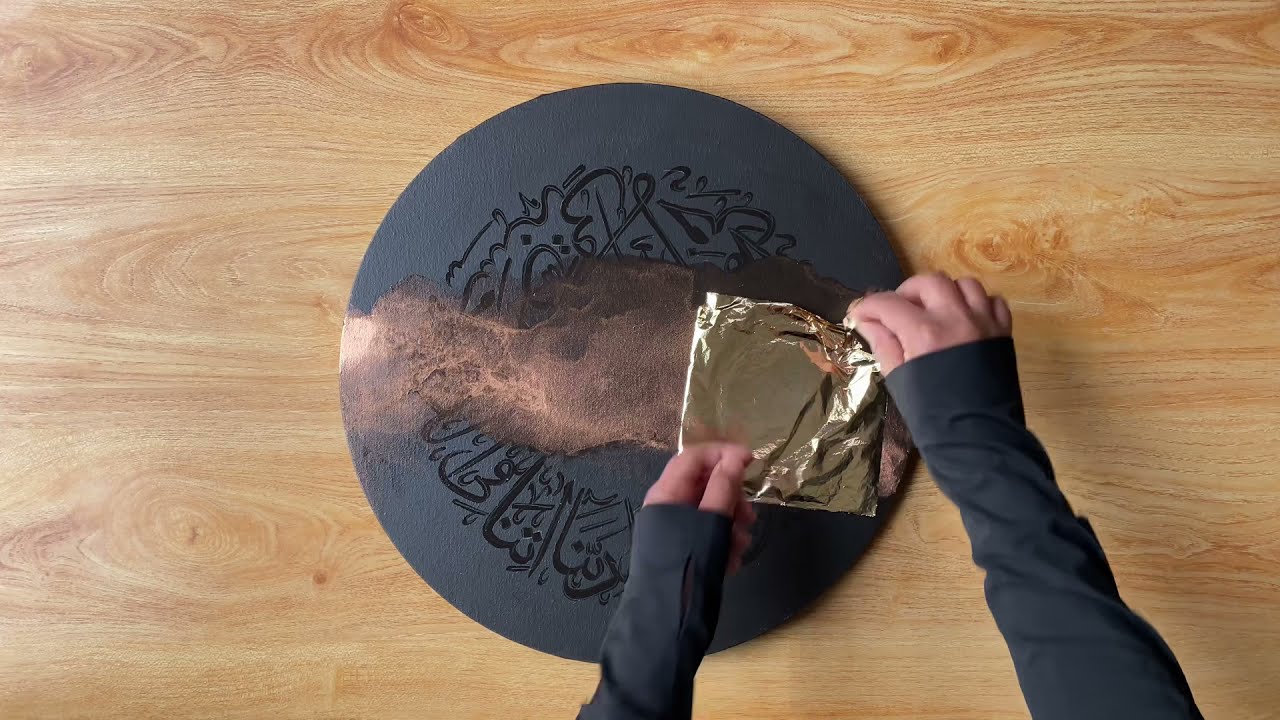An aerial shot captures a person with only their forearms and hands visible, clad in a long-sleeved black or dark charcoal shirt, meticulously working on a circular, black piece placed on a light brown wooden tabletop. The centerpiece of this metallic, shield-like object features intricate Arabic letters or ornate designs. The person is handling a sheet of gold foil, which they seem to be applying to or removing from a section of the piece that displays rusty, peach-colored discoloration or sand-like dust spread across its surface. The meticulous effort involves both hands holding a gold or silver wrapper, adding an aura of craftsmanship to the scene.